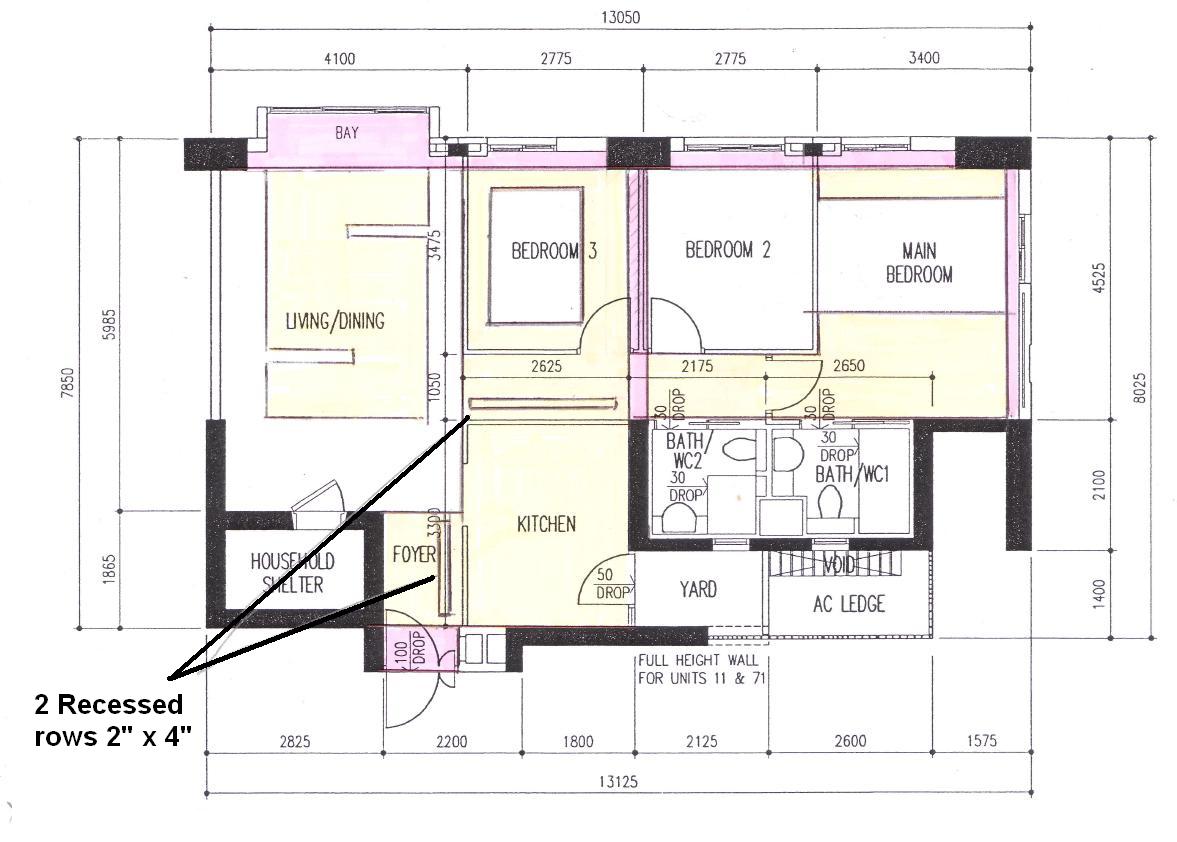The blueprint depicted showcases the architectural layout of a building. At the center, there is a spacious living and dining room area. Adjacent to this central area on the left side are Bedroom Two, Bedroom Three, and the Main Bedroom. These rooms are demarcated and filled with a subtle yellow shade, which accentuates their borders. Each bedroom, particularly the Main Bedroom situated towards the top, features a distinctive pink border indicative of window bays.

On the right side of the blueprint, beneath these bedrooms, lie Bathroom One and Bathroom Two. Adjacent to Bedroom Three is the kitchen, maintained within this consistent yellow-shaded area. Additionally, a household shelter is positioned in close proximity. Across from the living room, the foyer is also highlighted and fits cohesively within this layout.

Encircling the entire blueprint are various room measurements, characterized by black rectangular boxes that distinctly annotate the dimensions of each space. In the bottom left corner, there's a note stating "two recessed rows 2" x 4" (indicating feet). Black arrows extend to point out specific rectangular objects located in Bedroom Three and the foyer, providing further detail to these specific architectural features.